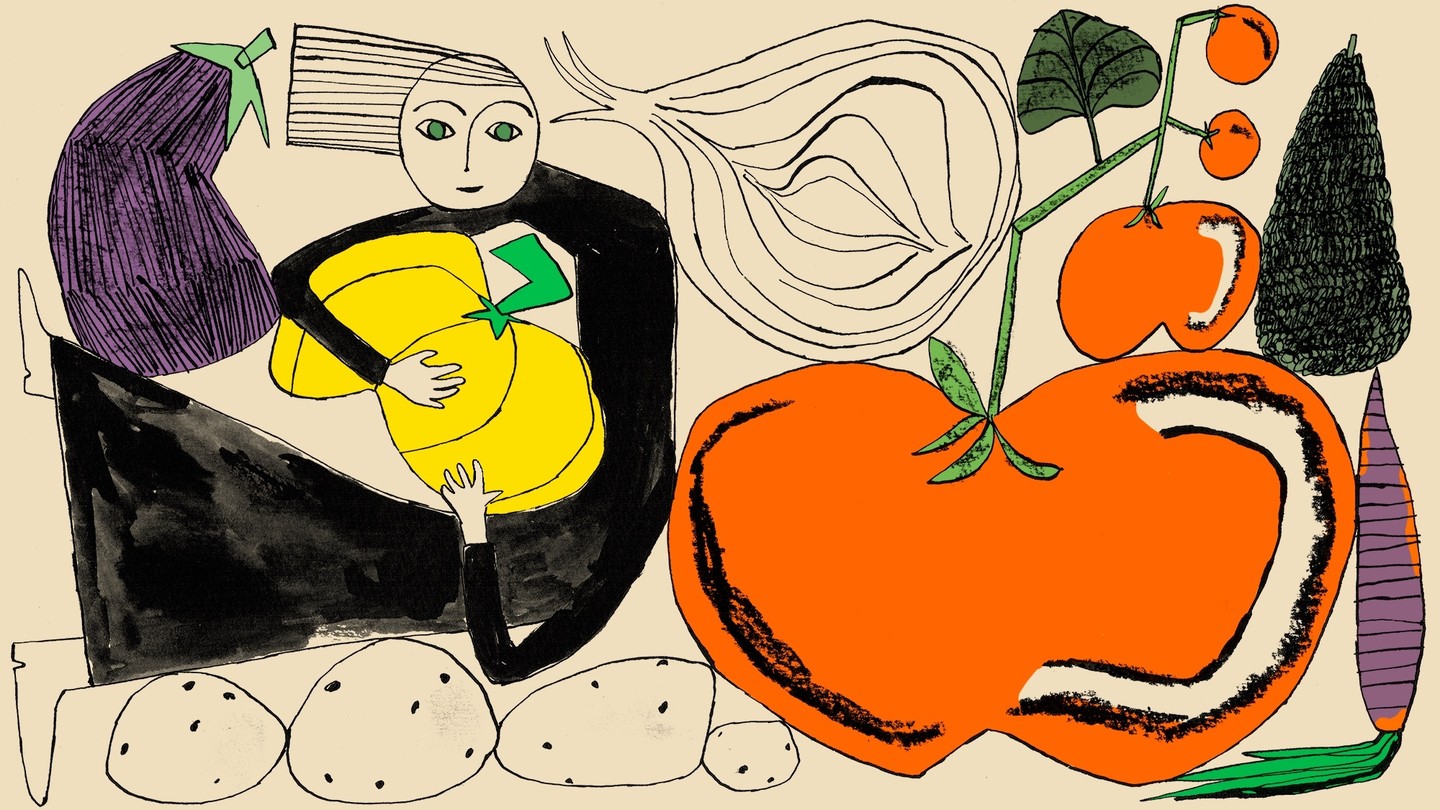This rectangular painting, notably much longer than it is tall, combines both detailed sketches and lively colors to illustrate a whimsical scene of fruits, vegetables, and a uniquely posed person. The person, with shoulder-length hair seemingly blown towards the left side of the image, curves their body in a backward C shape. Their feet point leftward while their torso curls around a large yellow pumpkin with a green stem, enveloped by their exaggeratedly long arms and legs. They have striking green eyes and wear a simple black dress. The background features a delightful assortment of produce, including an eggplant, a cut-open onion, tomatoes, a purple carrot, and potatoes, upon which the person is partially reclined. Additionally, there are other vibrant and uniquely shaped fruits and vegetables, such as oranges, and several sketchy outlined items, some black-coned and others circular with dots, enhancing the painting's charmingly childlike and detailed aesthetic.